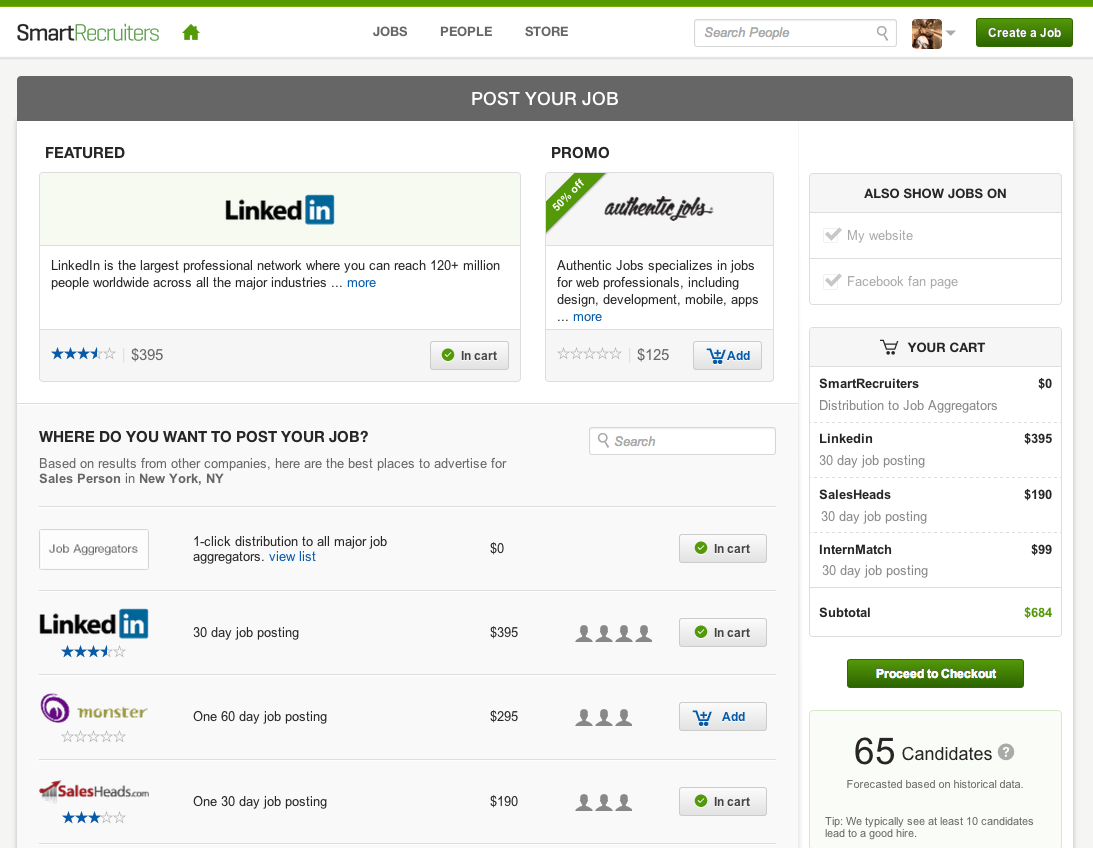The image showcases a recruitment website designed for sourcing candidates for various job roles. At the top of the page, the logo "SmartRecruiters" is prominently displayed with "Smart" in black and "Recruiters" in green, accompanied by a small green house icon. The top middle section features navigation tabs labeled "Jobs," "People," and "Store." On the far right, there is a search bar specifically for people, allowing users to search for individuals. Adjacent to the search bar, a green button with white text invites users to "Create a Job."

Below the header, a grey strip spans across the screen with the text "Post Your Job" in white. Further down, the page highlights LinkedIn as a featured platform, noting it as the largest professional network, capable of reaching over 120 million people globally across major industries.

A promotional section indicates a 50% discount on "Authentic Jobs," while a section titled "Where do you want to post your job?" provides recommendations based on results from other companies for a salesperson role in New York. The recommended platforms include LinkedIn, Monster, and saleshead.com, each with specified job posting durations: 30 days for LinkedIn, 180 days for Monster, and 30 days for saleshead.com.

The cost breakdown for advertising on these platforms is also provided: LinkedIn at $395, currently added to the cart; Monster at $295, not in the cart; and saleshead.com at $190, also in the cart. The current total cost for the selected services is displayed as $684.